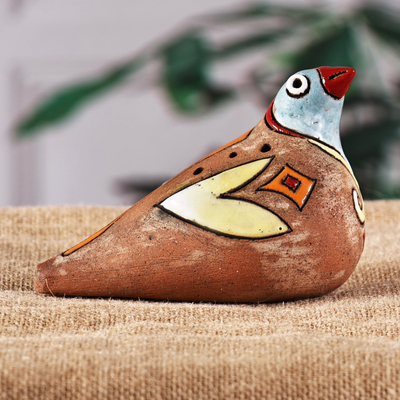A detailed photograph captures a meticulously crafted pottery figurine of a bird, perched gracefully on a textured, upholstered surface. The upholstery features a Sahara sand base color adorned with subtle, pale yellow sand-colored details, adding depth and warmth to the setting. In the slightly blurred background, a white wall contrasts softly with the suggestive green leaves of a plant, providing a calm and natural ambiance.

The bird figurine is oriented with its tail pointing to the left and its head, breastbone, and beak angled towards the top right corner of the image. Its head is uplifted, giving the bird an alert and inquisitive appearance. The bird's body is predominantly painted in a rich brown, with an artistic, slightly squished heart-shaped yellow wing on its side. Nestled within this yellow wing is an orange diamond, further detailed with a small red square at its center. Three black dots accentuate the area above the yellow wing, adding texture and intrigue.

The bird's head is painted a delicate light blue, juxtaposed strikingly with its red beak. An expressive, large white eye with a black dot gives the bird a characterful and lively look, making the figurine both charming and captivating.